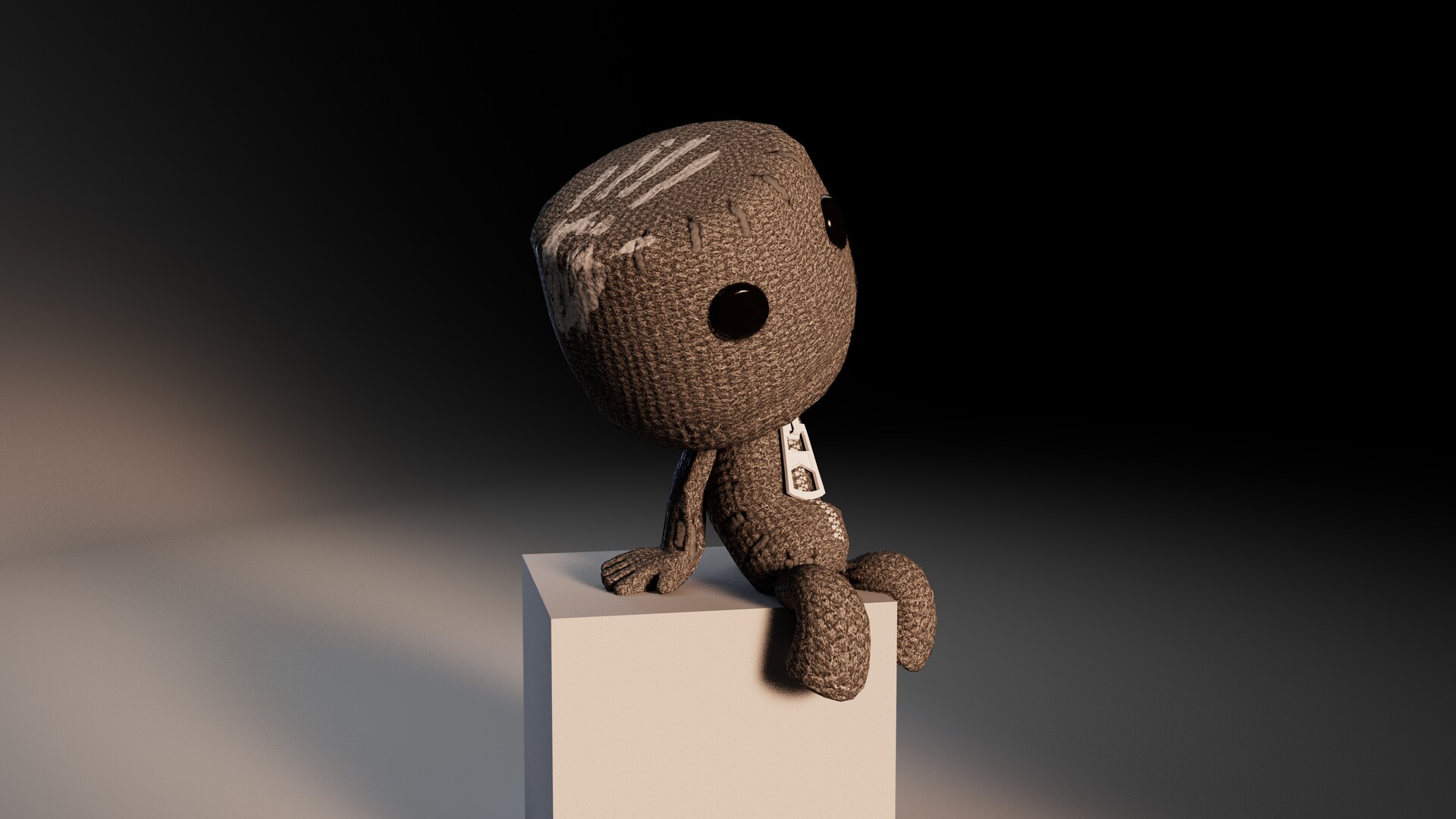This image is a horizontally aligned rectangular digital screenshot of a 3D render featuring a character resembling the one from LittleBigPlanet on PlayStation games. The background is a gradient mix of light gray and dark gray at the bottom, transitioning to solid black in the upper right corner and across the upper left side. The character is a small, knitted stuffed figure with a medium brown, bag-like material and two black button eyes. It has a round, slightly flattened head with a distinctive white handprint partially covering the top and side. The figurine has a narrow body with a zipper that runs from its neck down to its belly, and it rests its little arms on a white, cubicle-shaped stand upon which it sits. The bottom of the stand is out of the frame, and both it and the character cast visible shadows.